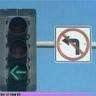A highly detailed, close-up image showcases a gunmetal-colored stoplight mounted on a silver pole. The green arrow on the stoplight is illuminated, indicating the direction to proceed. Adjacent to the stoplight, there is a prominently displayed white square sign with a black border. This sign features a black arrow with a red circle and a slash mark through it, signaling a prohibited action in that direction. At the bottom of the image, a very narrow lavender strip with indistinguishable black text is visible. Although the font can't be read due to the small size of the image, the clear blue sky in the background suggests it is daytime. The image appears slightly pixelated and grainy, likely due to significant zooming in, yet it remains of excellent quality overall.